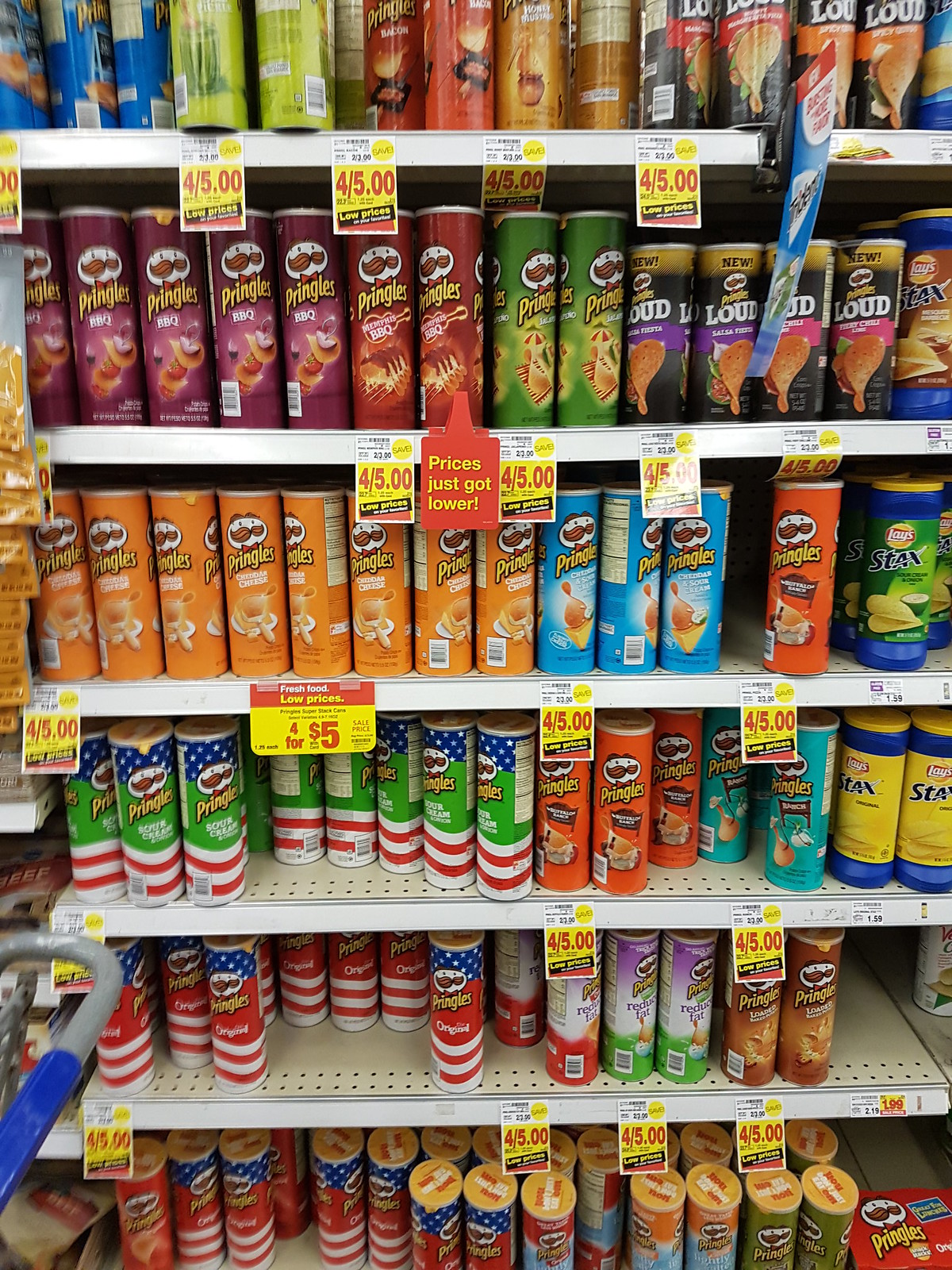The photograph depicts a grocery store display of Pringles potato chips arranged on six white shelves, each punctuated with two rows of circular holes along the edge. Each shelf holds around 15 canisters of Pringles, showcasing a wide variety of flavors and colorful packaging. The top shelf features canisters in red, green, and various colors. Moving down, the second shelf displays Pringles in vibrant orange, blue, and dark blue canisters. On the third shelf, the cans are adorned with red, white, and blue stripes, green, and a mixture of blue, white stars, orange, aqua, and yellow. The fourth shelf has canisters in red, white, and blue, and a combination of purple, white, green, orange, and brick colors. At the bottom, more canisters in red, white, and blue, along with various other colors, can be seen. Each shelf end is marked with yellow price tags, most of which advertise a deal of four cans for five dollars.